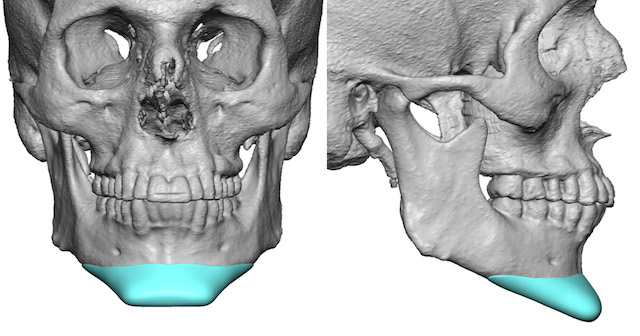The image depicts two digitally rendered skulls, seemingly created using a 3D graphics program or derived from a scan. The skull on the left is oriented to face directly forward, making eye contact with the viewer, whereas the skull on the right is shown in profile, highlighting its right side. 

Both skulls feature a light blue section highlighting their chin areas, giving a subtle but distinct coloration to this specific region. The chin of the left skull appears notably wide and somewhat pointy, while the chin of the right skull is extremely pointed, angling downward in an unnaturally sharp manner.

Details such as the teeth, jawlines, and eye sockets are visible in both skulls. However, the nasal area of the left skull appears slightly irregular or deformed. This meticulous rendering captures the eerie intricacies and unique characteristics of each skull, enhancing the overall surreal and scientific aesthetic of the image.